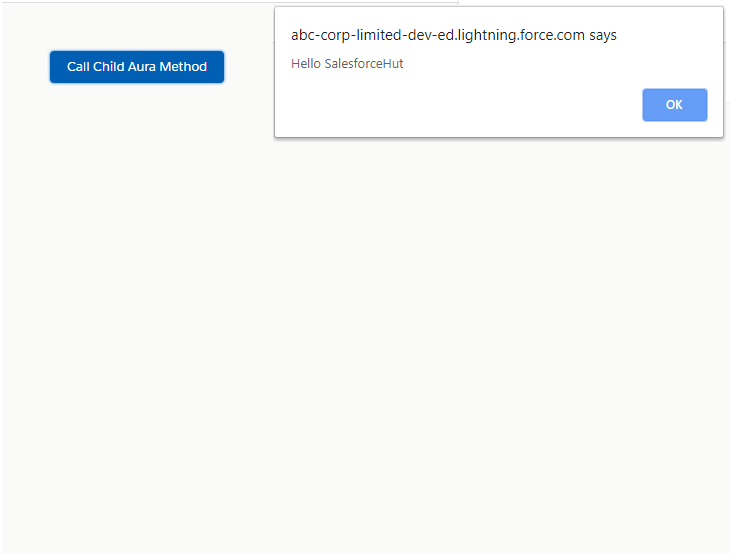The image features a large, prominent blue box dominating the scene. Within this larger blue box, there is a smaller, darker blue box that contains the text "call child aura method." Below this, another large element stands out: a white box bordered by a blue outline. This white box displays the text "ABC Corp limited dev ed dot lightning dot force dot com says hello Salesforce." Near the lower right corner of the white box, there is a conspicuous blue button labeled "OK." Additionally, in the upper right corner of the image, a small visual search icon resembling a blue camera lens can be observed.